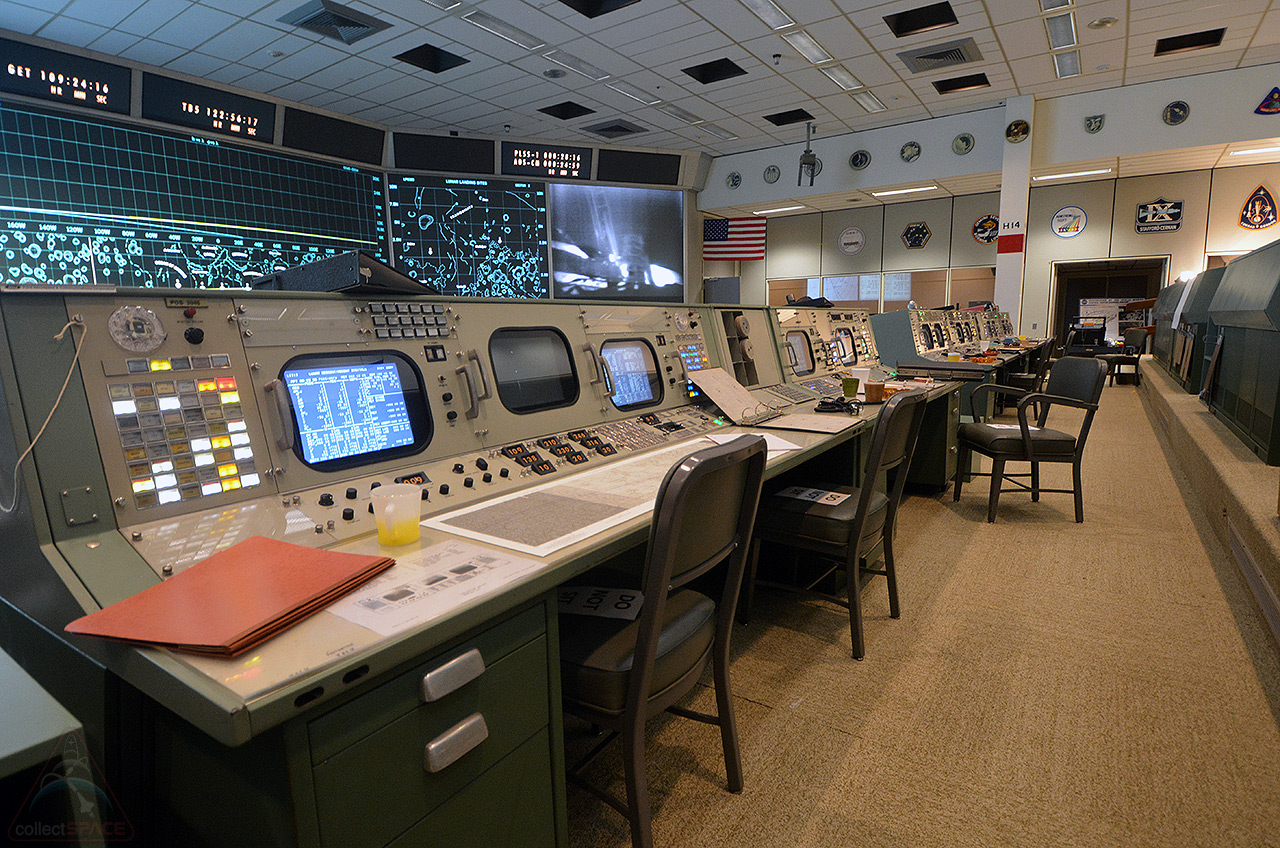The image depicts a command center, possibly a NASA control room, filled with an array of technical equipment and indicative details. Central to the room is a series of large electronic boards and screens, some displaying grid-like patterns and flight paths reminiscent of an air traffic control environment. In the backdrop, an American flag hangs prominently, adding a patriotic touch to the otherwise utilitarian setup. 

In the foreground, a row of desks, each outfitted with multiple monitors, buttons, and knobs, spans the room. Some of these desks have metal chairs with gray cushions, three of which bear white signs reading "Do Not Sit." There are various items scattered across the desks, including file folders, three-ring binders, and cups, one of which contains a half-filled plastic container of orange juice.

The room’s background features additional screens and a wall adorned with what seem to be awards or achievements. Notably, there is a picture of an astronaut on the moon, reinforcing the aerospace theme. Bright natural lighting illuminates the room, accentuating the clear and organized layout of this high-tech command center. The flooring is covered with a gray rug, grounding the space in a neutral palette. No people are visible in the image, emphasizing the stillness and focus of the environment.